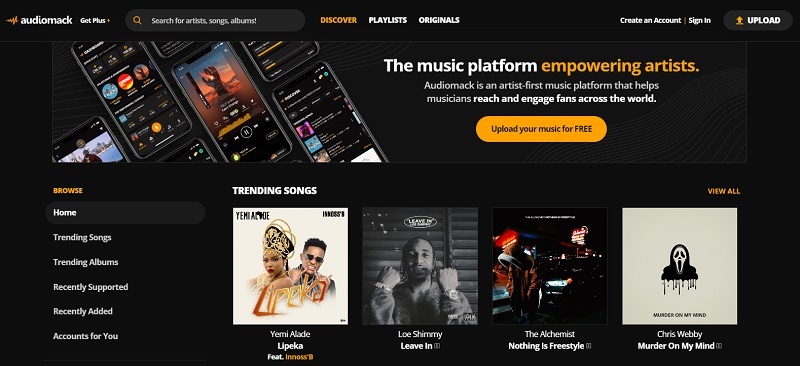The image showcases the interface of the Audio Mac platform. At the top left corner, the logo "Audio Mac" is displayed against a black background. The main search bar prompts users to "search for artists, songs, and albums." The "Discover" tab is highlighted in orange, alongside other tabs such as "Playlists" and "Originals." 

On the right section of the interface, options like "Create an Account," "Sign In," and "Upload" are visible. Centered prominently on the image is the tagline, "The Music Platform Empowering Artists," with "Empowering" and "Artists" highlighted in orange. Below this slogan, it is explained that Audio Mac is an artist-first music platform designed to help musicians reach and engage fans worldwide.

Beneath this description, there is an elongated orange box with rounded edges labeled "Upload Your Music for Free." Surrounding this box, several smartphone screens with various displays are shown, including a picture, a list, and a series of profile pictures.

At the bottom part of the interface, the "Browse" tab is highlighted in orange. Additional category tabs include "Home," "Trending Songs," "Trending Albums," "Recently Supported," "Recently Added," and "Accounts for You." Within the "Trending Songs" section, the image features album covers of trending songs such as "Lipica" by Yuri Adel, "Slavery," "Leave In," "The Algernist," "Nothing is Freestyle," and "Murder on My Mind" by Chris Webley.